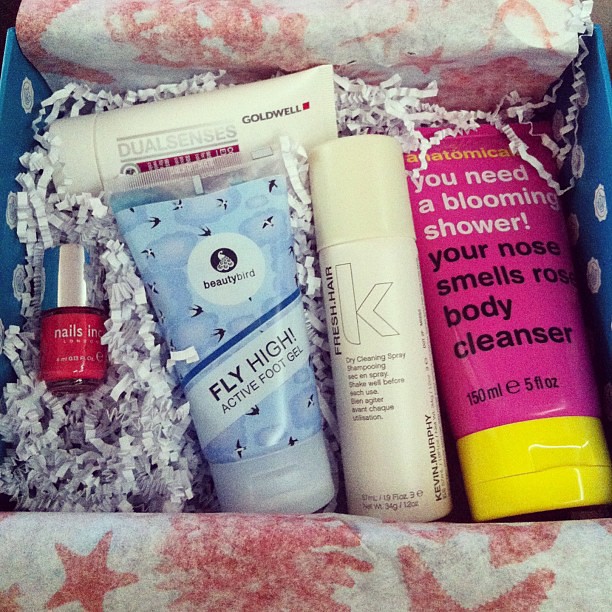The photograph features an elegantly arranged gift box filled with an assortment of bath and beauty products. The box, which has blue walls and is lined with an intricately designed tissue paper adorned with pinkish-peach starfish and coral patterns, contains a variety of items cushioned by crimped white paper strips. 

Inside the box, starting from the right, there is a prominent pink tube with a yellow cap labeled "Anatomicals - You Need a Blooming Shower, Your Nose Smells Rosy Body Cleanser." Next to it is a light tan cylinder marked as "Fresh Hair K - Dry Cleaning Spray Shampoo." Further to the left, a blue tube of "Beauty Bird - Fly High Active Foot Gel," decorated with bird illustrations, adds a touch of serenity. Centrally positioned in the box, there is pink nail polish with a silver cap, branded as "Nails INC London." 

At the top left corner, a white tube named "Dual Senses by Goldwell" can be seen, although some of its text is obscured. The items are neatly laid out, enveloped in both white and red tissue paper, which enhances the festive presentation. This intricate display suggests that it is either a curated gift set or a beautifully packaged purchase from a premium store.